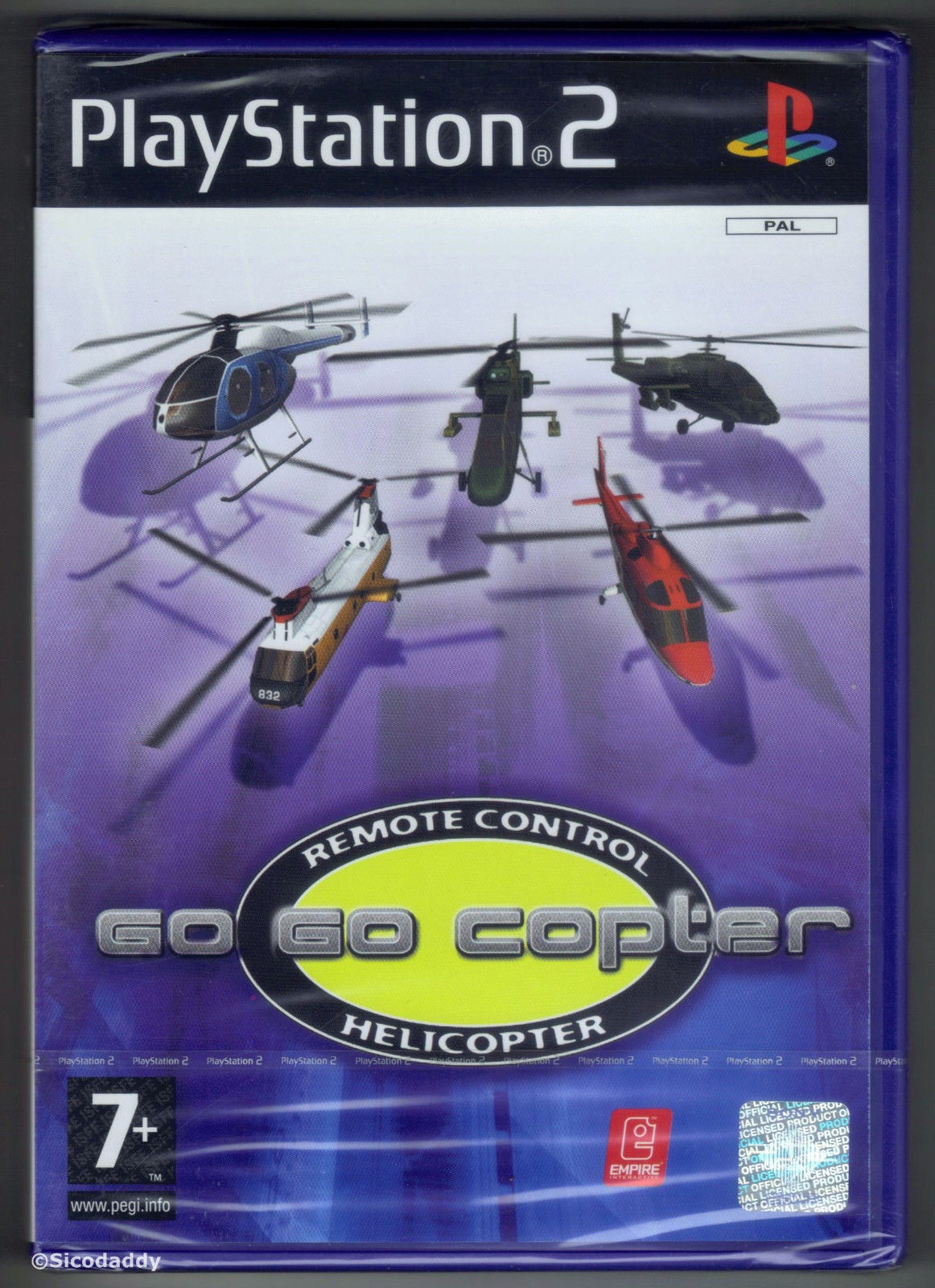The cover of a PlayStation 2 game, titled "Go-Go Copter: Remote Control Helicopter", features prominently on a typical dark blue case. At the top of the cover, "PlayStation 2" is written in white text within a black bar, accompanied by the multi-colored PlayStation logo to the right, with "PAL" noted underneath. The middle section of the cover shows a vivid and dynamic scene with five digitally-rendered remote control helicopters of varying colors, shapes, and sizes, flying over a purple background. The title "Go-Go Copter" is displayed in gray lettering towards the bottom, set against a bright yellow and black landing pad-like oval shape. Additional details include a notification on the bottom left stating the game is suitable for ages 7 and up, a small foil seal, and a copyright watermark, “Sicko Daddy,” in the bottom left corner. Further down on the right side are two smaller logos, one red and one silver.